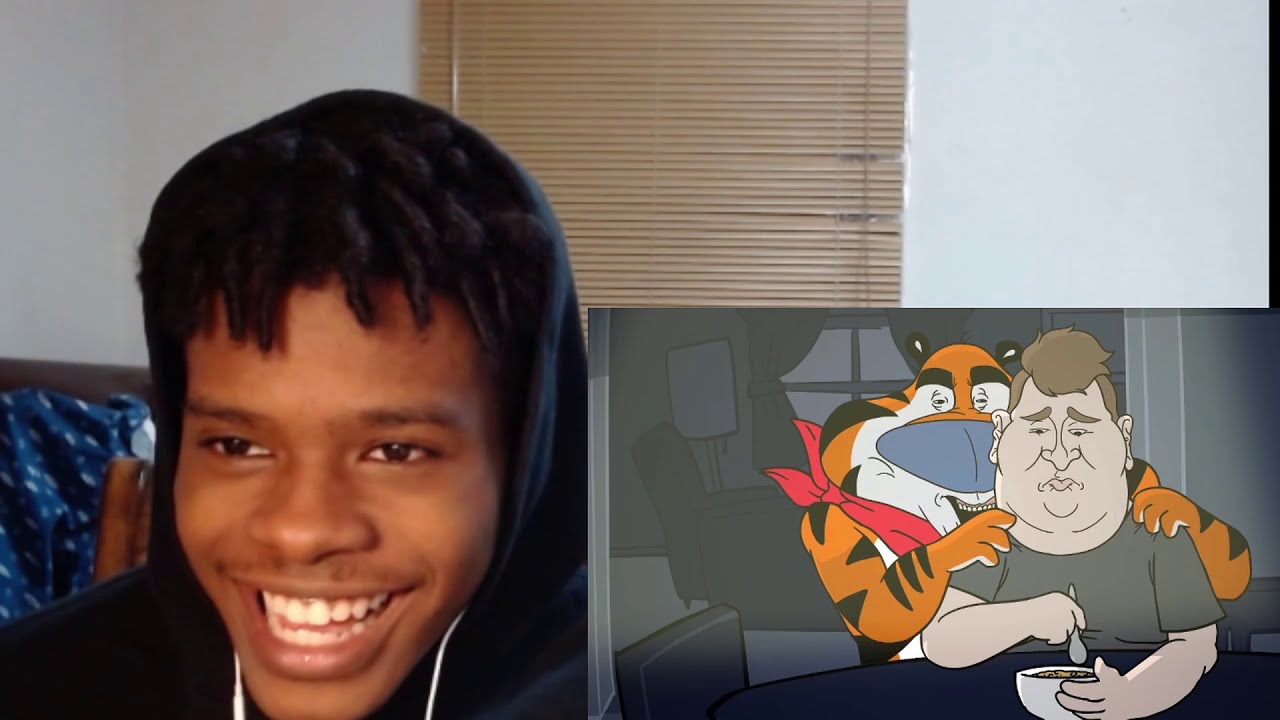In this image, a young dark-skinned boy is sitting in his room, smiling broadly with a visible display of his teeth. His black hair is styled in tiny curls atop his forehead, and he's wearing a dark blue hoodie. The background features a white-colored wall with closed brown curtains or blinds. On the lower right corner of the image, there's an edited overlay of a cartoon scene depicting Tony the Tiger massaging the shoulders of a pudgy Caucasian man unhappily eating a bowl of cereal at a table. Tony the Tiger has a mischievous expression on his face. The boy appears to be laughing, presumably at the humorous cartoon next to him. On the left-hand side, there's a hint of a blue chair or material in the scene.